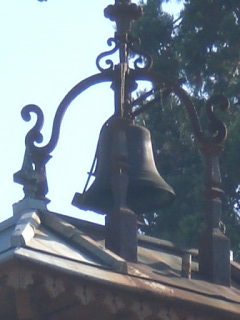This photograph features a very old, vintage bell with a unique external ringing mechanism mounted on an aged wooden roof. The dark brown bell, crafted from thick, cast iron material, is mounted on an elegant metal arch frame made of decorative, hammered ironwork, featuring swirling, curly-Q designs at the top. The distinctive mechanism includes an external hammer suspended on a hinged apparatus, allowing a rope to be pulled to tap the outside of the bell. The roof, displaying signs of aging, is adorned with intricate wood carvings under the fascia and beams, adding to the vintage charm. In the background, a tall pine tree with thick green leaves reaches upward against a hazy blue sky. The photograph, though cropped and not capturing all surroundings, showcases the craftsmanship and timeless beauty of this historic bell and its picturesque setting.